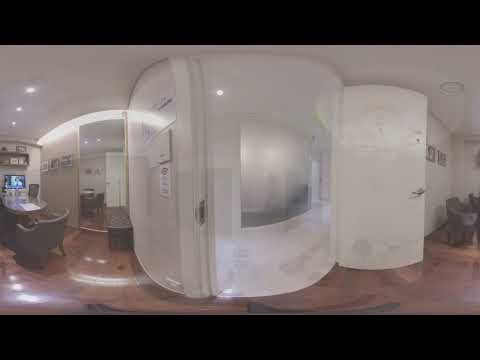The image showcases the interior of a house or possibly an office building, captured with a fisheye lens that distorts everything into a super round and curvy appearance. The floor is a glossy, shiny brown wood, contrasting with the uniformly white walls and ceilings. On the left side of the image, a rounded gray chair is pulled up to a desk that has a computer monitor on it. Adjacent to the desk is a small brown bench. A wall displays three organized portraits, and a paper certificate hangs nearby. Centrally, a large, white, rectangular pod with an open door suggests a space for sitting or working but appears empty inside. LED spotlights are lined up in a horizontal pattern on the ceiling. The right side of the image shows more chairs, some lined up against the wall, and a shelf with two sections holding various items. A possible window or mirror reflects some of the room's details, amplifying the warped, interconnected images effect. Two white doors lead into different parts of the building, one transitioning into an unseen hallway.